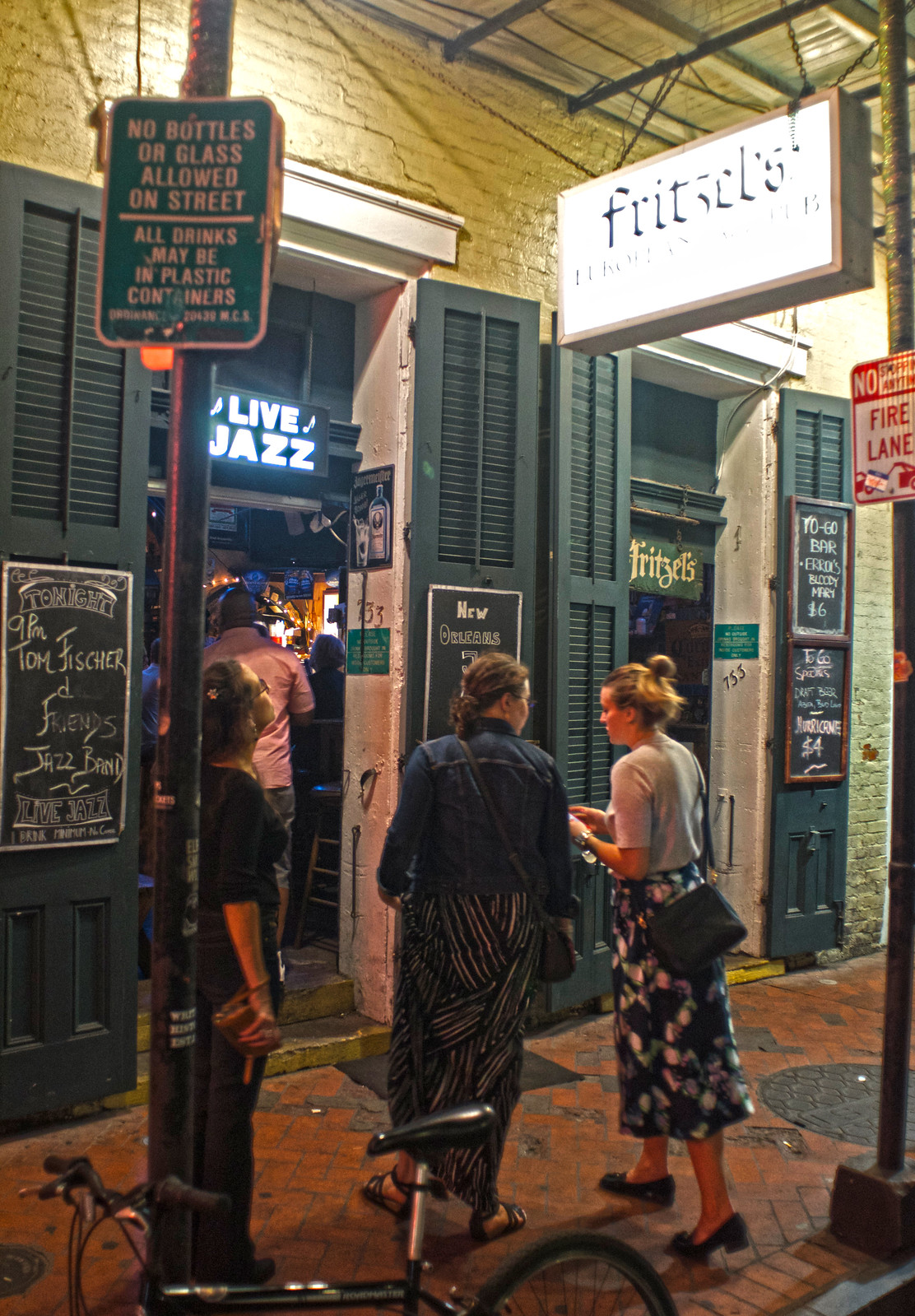The photograph, a color image in portrait orientation, captures a detailed street scene outside Fritzels, a bar marked by a white rectangular sign with black script lettering reading "FRITZELS" and a neon sign above the entrance proclaiming "LIVE JAZZ." Three women stand on an orangey-red brick or stone walkway. The two women on the right engage in conversation. The woman on the far right wears a short-sleeved gray shirt, a flowered skirt, and carries a black shoulder bag; her blonde hair is pulled up. The woman beside her sports a denim jacket, a black and white skirt, and a purse slung over her left shoulder. To their left, another woman, with her back against a pole, gazes up at the Fritzels sign. This pole bears a green sign declaring, "No Bottles or Glass Allowed on the Street, All Drinks May Be in Plastic Containers." The entrance behind them is adorned with four dark green shutters, two on either side of a double door, each door topped with relevant signage – "LIVE JAZZ" on the left door and "FRITZELS" on the right. Chalkboard signs hang from the shutters, adding to the charm of the scene. In the foreground, a bicycle is propped against the pole, and to the far right, a separate pole reads "No Parking Fire Lane." A noticeable crack runs along the brick building's facade, contributing to its vintage ambiance.